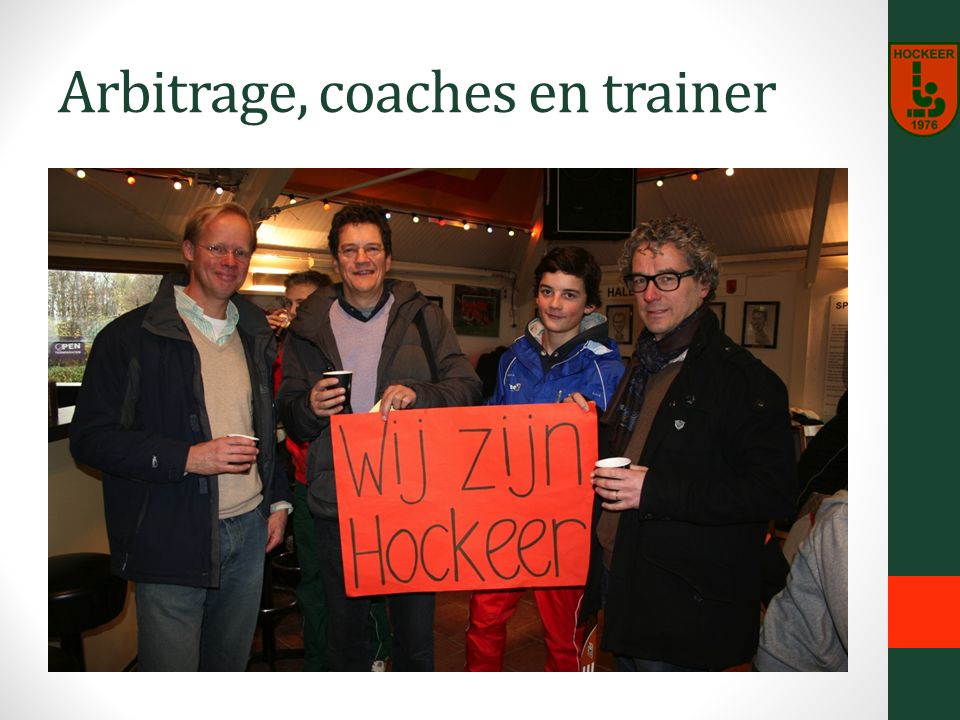The image depicted in the photograph has a white border with green text at the top, stating "Arbitrage Coaches and Trainer," despite minor variations in wording provided by different observers. This photograph is likely part of a poster or a slide from a presentation due to its overall composition and layout, reminiscent of a PowerPoint slide. The right side of the image features a vertical green stripe with a red square toward the bottom and a red, shield-like logo at the top reading "Hockeyer 1976."

The main focus of the photograph is four individuals—three men and one boy—smiling and holding a bright orange poster with writing in an unspecified foreign language. The subjects are indoors, dressed warmly in coats and heavy clothes, indicative of a cold environment. The background reveals white walls adorned with numerous pictures and a window, suggesting they are in a well-decorated room or office space. The colors in the image include a range of tan, red, orange, blue, black, white, and gray, contributing to its vibrant yet professional feel.